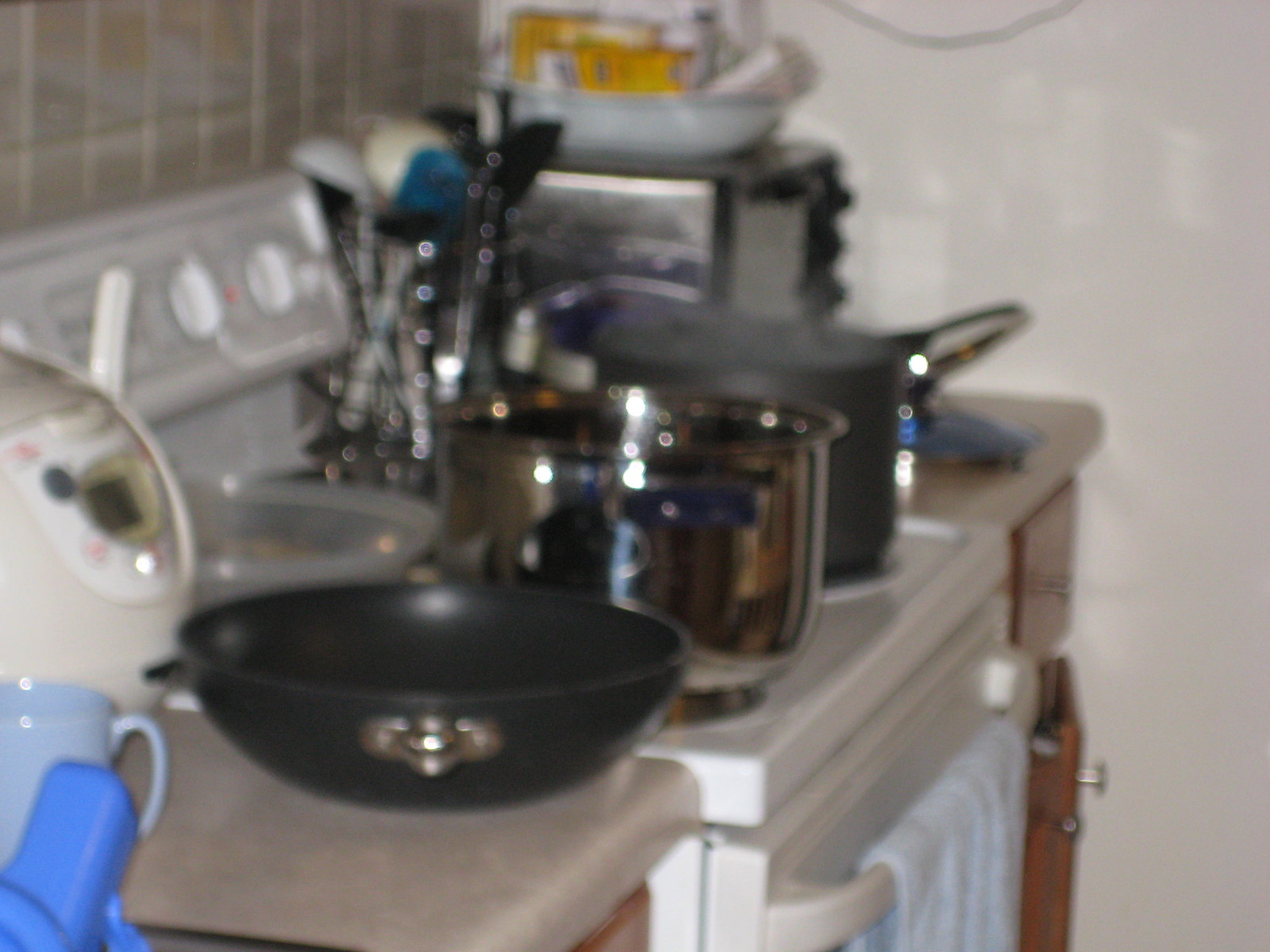The photograph captures a bustling kitchen scene, predominantly concentrated on the left side of the frame. Dominating this area are two brown kitchen cabinets adorned with silver knobs, flanking a central white stove. The stove is busy with various pots: a silver pot with black handles occupies the lower left burner, while a black pot with silver handles sits on the right burner. Despite the image's overall blurriness, a wire cylinder filled with kitchen utensils is discernible. To the lower left, a black pot with a small silver handle rests on the countertop, adjacent to a device that appears to be a bread maker. A light blue towel drapes from the white oven handle, adding a splash of color. The backsplash behind the stove is a creamy tile, contrasting with the white walls of the kitchen. Overall, the scene exudes a homely, lived-in atmosphere.